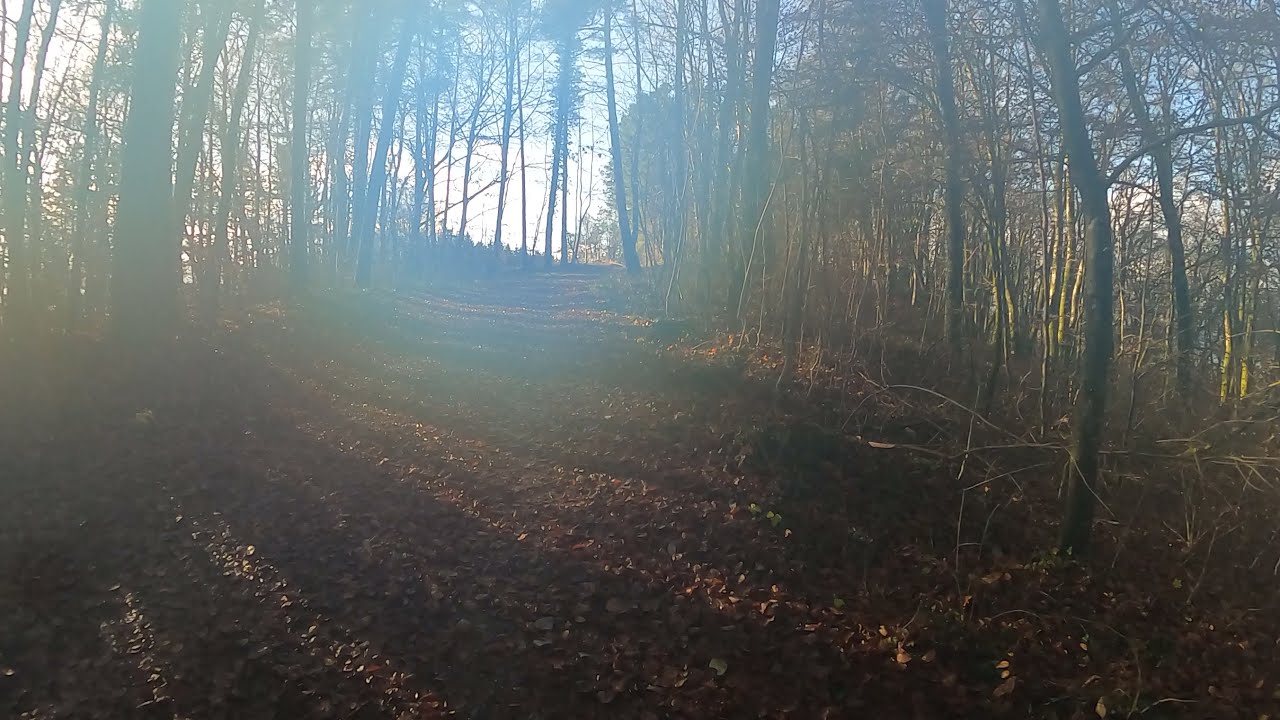The image depicts a serene mountain trail winding through a dense, forested area. The pathway, approximately four to five feet wide, is predominantly covered in brown gravel and fallen autumn leaves. A sense of tranquility is enhanced by a light mist or fog that pervades the scene, likely a result of the sun shining through the trees from the left-hand side. This sunlight casts long, intricate shadows and a radiant glow, creating a subtle halo effect that adds to the overall haziness.

The forest consists of numerous skinny, dark gray tree trunks that are curved and mostly leafless, though some trees in the background retain their foliage. These trees line both sides of the path, and the majority are bare, accentuating the season's autumnal shift. The scene captures the essence of a quiet, secluded trail, with no visible objects or people, framed by a backdrop of a blue sky softly veiled by clouds. The upward slope of the trail and the slight bend of some trees on the right-hand side contribute to an impression of depth, indicating a path that ascends through this idyllic woodland landscape.